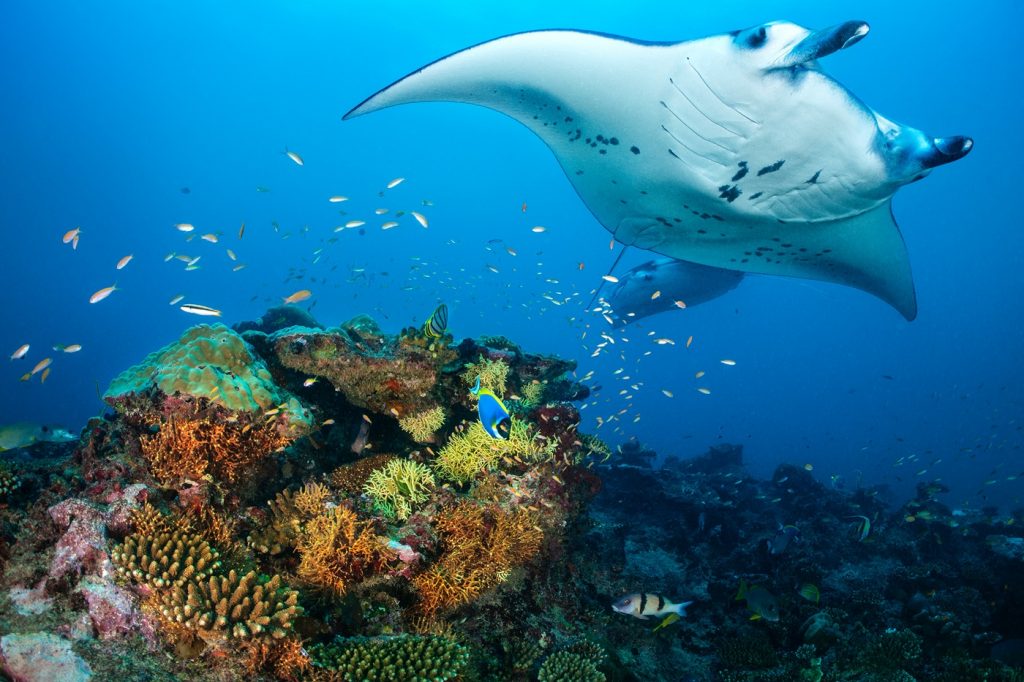In this captivating underwater photo, the main focus is a majestic stingray gliding through an endless blue sea from right to left. The stingray’s blue top contrasts with its white underbelly, which bears visible gills and eyes, while its unique claw-like appendages add an intriguing detail to the scene. Below the stingray, in the bottom left of the image, a vibrant coral reef bursts with colors including browns, greens, turquoise, orange, yellow, and pink, illuminated by a camera flash. Around the glowing coral, a swarm of small fish, possibly anchovies or sardines, swim energetically, their silvery and blue hues shimmering against the marine backdrop. The overall scene artistically captures the dynamic and colorful underwater ecosystem.